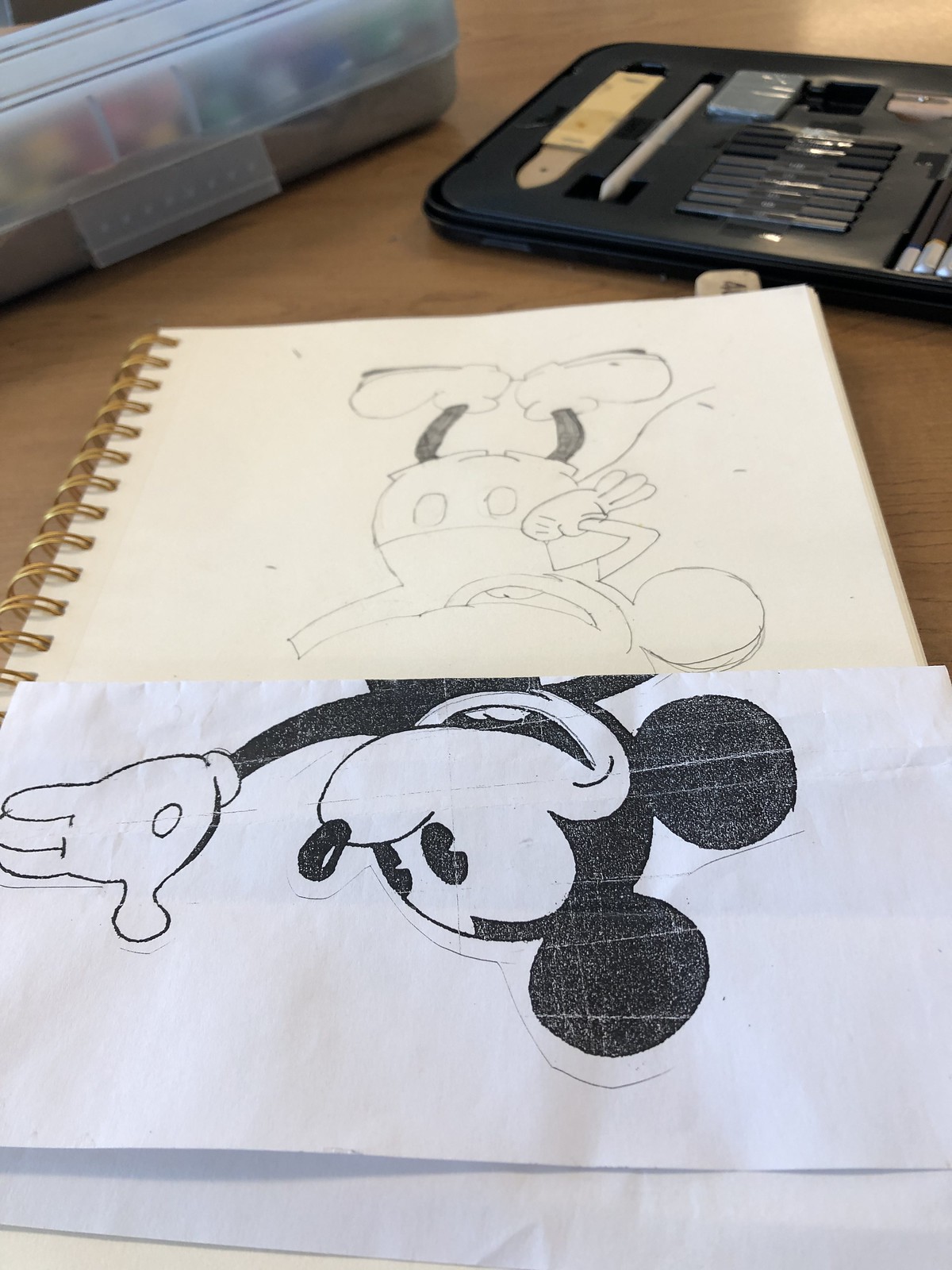The image captures a cluttered wooden table surface adorned with various artistic tools and materials. At the center, there is an upside-down spiral-bound sketchpad displaying an incomplete, uncolored outline of Mickey Mouse, sketched in pen or pencil. The only shaded sections of the drawing are Mickey's legs. Partially covering the lower half of the notebook, including Mickey's head, is a folded sheet of paper printed with another image of Mickey Mouse.

Positioned towards the top of the frame, several art supplies are scattered. A black plastic art kit is open, revealing charcoal pieces, a white smudge pen, an eraser, and some other flat, rectangular objects. In the top left corner of the image, a transparent plastic container, possibly a storage bin, is visible. It is closed but reveals a variety of colorful items inside, likely markers or colored pencils. The arrangement and variety of materials suggest an ongoing artistic project in progress.